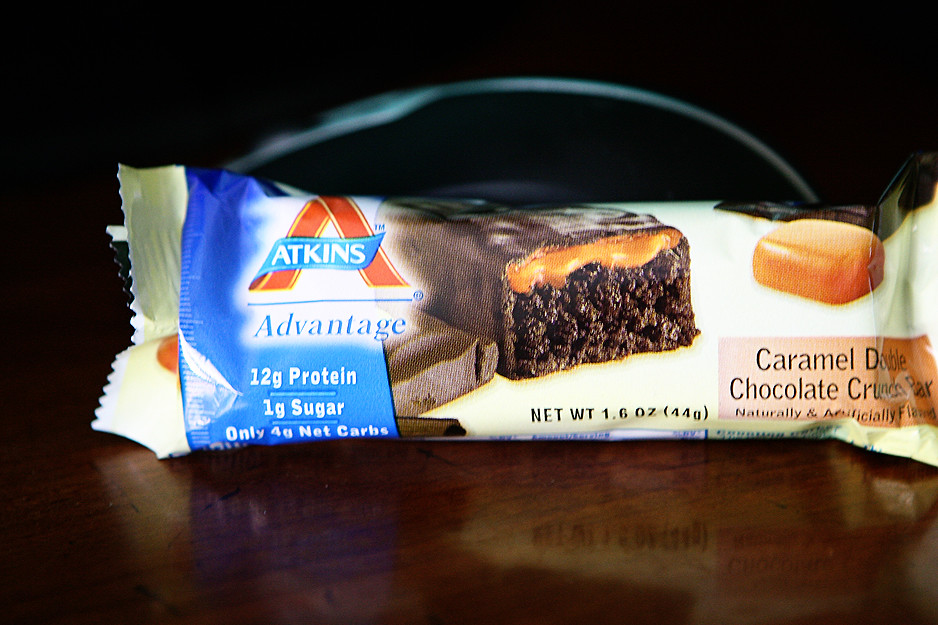The image showcases a close-up view of an Atkins Caramel Double Chocolate Crunch Bar. The bar is prominently positioned, highlighting its layers; the chocolate coating is visible at the forefront, topped with a luscious layer of caramel cream. On the right side, a smaller piece of caramel is displayed, illustrating the rich texture. To the left of the bar, the bright red Atkins logo is prominently featured, consisting of a bold "A" with the word "Atkins" in white letters set against a blue ribbon. Below the logo, the word "ADVANTAGE" is written in blue. In smaller print, nutritional information indicates that the bar contains 12 grams of protein and just 1 gram of sugar. The background is black, creating a striking contrast that makes the caramel and chocolate hues more vibrant, and a brown table provides a rustic base for the arrangement.